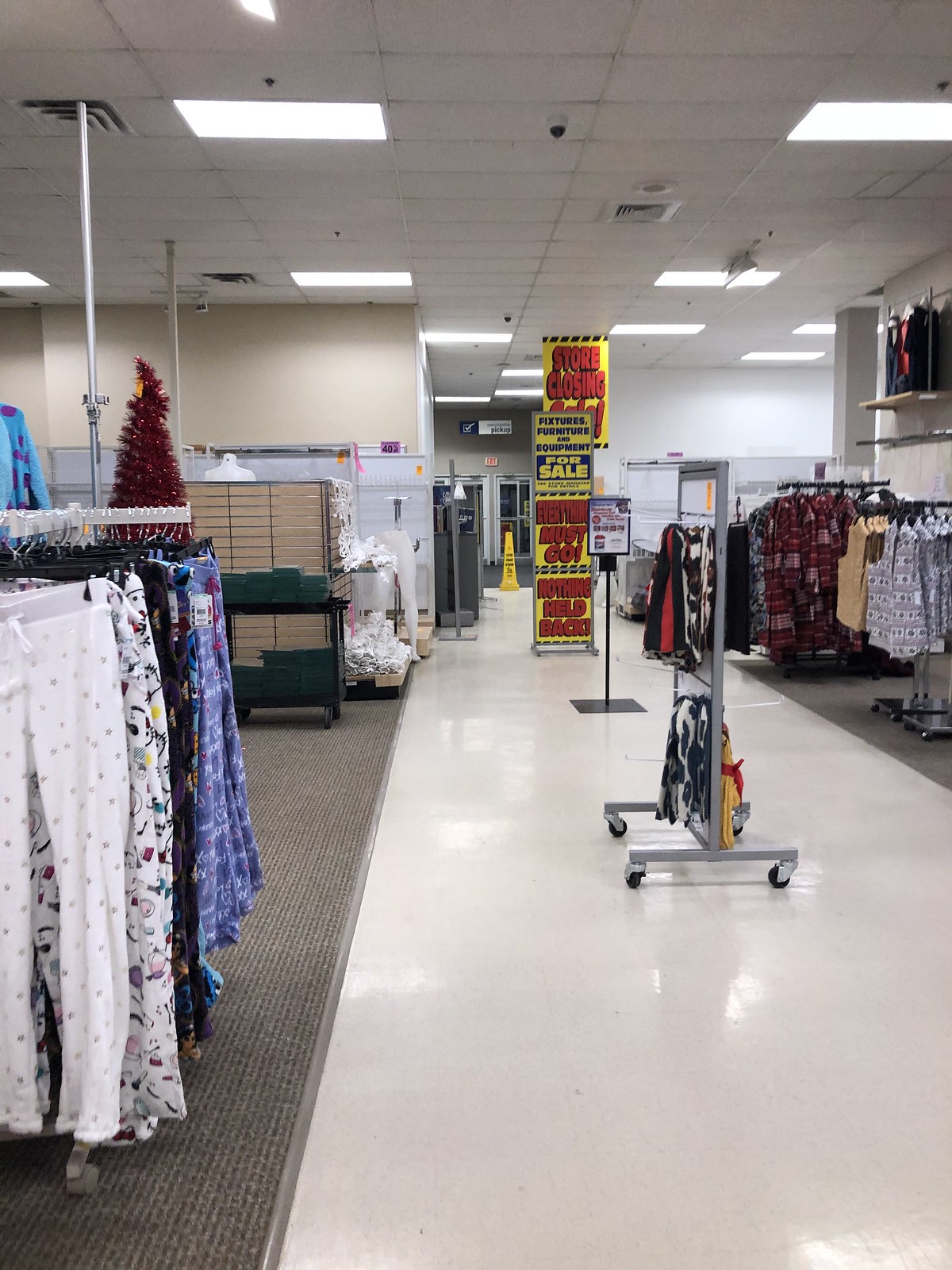In this rectangular photograph, taken from the perspective of standing in a store, we're looking down a brightly-lit aisle. The aisle is flanked by rounders of clothes on both the left and right sides. The floor is a shiny white linoleum, which contrasts with the carpeted areas beneath the rounders.

On the left side of the aisle, the rounders display a variety of colorful pants, possibly sweatpants or sleepwear, distinguished by their vibrant prints. Situated further back on this side, a striking red Christmas tree adds a festive touch to the scene. On the right, the rounders are adorned with an assortment of women's sleeveless shirts or vests, with red plaid robes visible further down.

The store's drop ceiling is adorned with fluorescent lighting, casting a bright, uniform light over the entire scene. In the center of the aisle, several bold signs hang from the ceiling and stand on the floor, bearing urgent messages in yellow, red, and black text. The signs announce a "Store Closing Sale," with details outlining that furniture, fixtures, equipment, and everything else must go, emphasizing that nothing will be held back. Customers can see that these signs stretch towards the back doors of the store, directing them where to go for further deals.